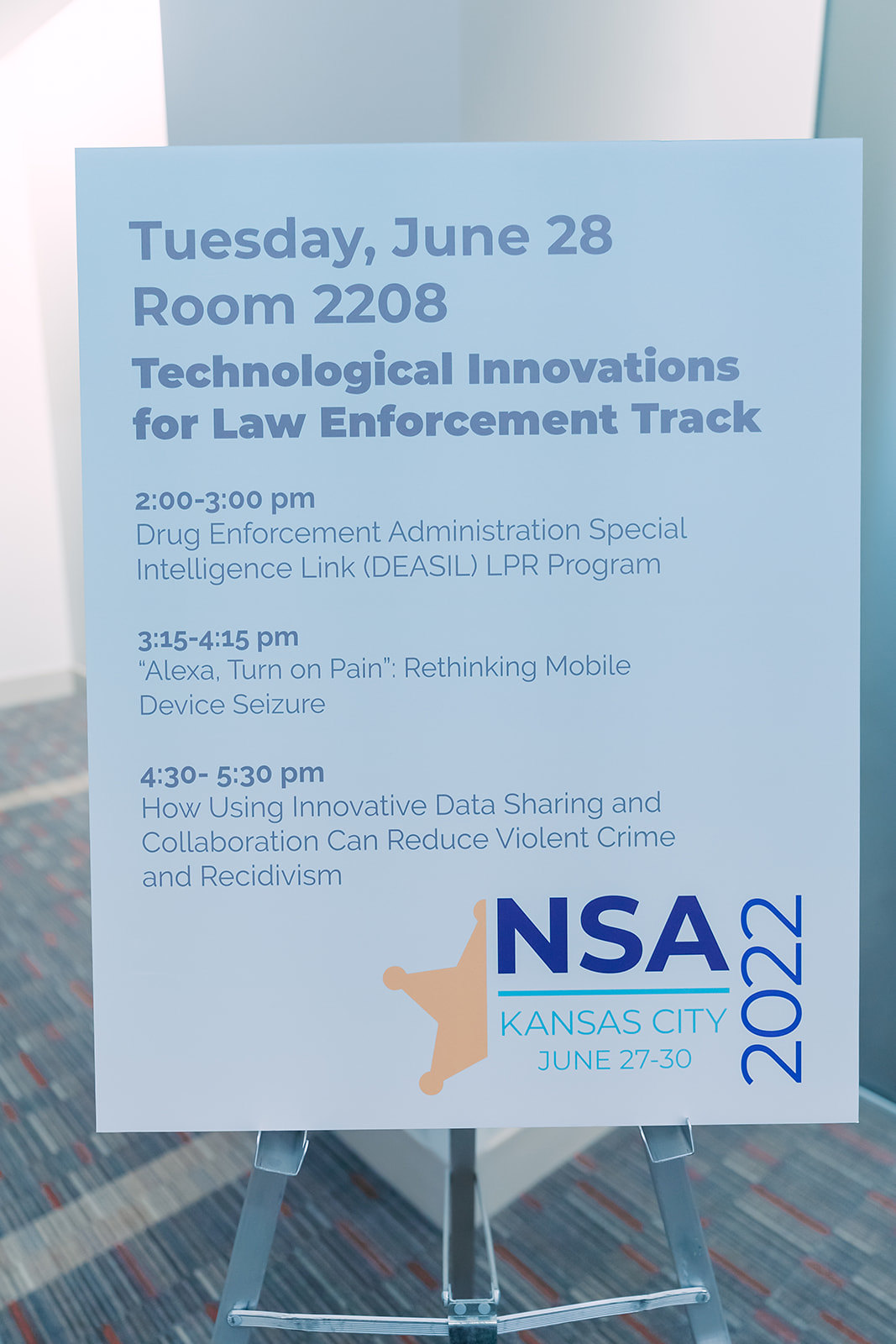The image depicts a detailed itinerary board on an easel outside a conference room, possibly in a hotel, for a series of presentations under the "Technological Innovations for Law Enforcement Track." The background of the sign is white, and it is dated Tuesday, June 28th, with the location specified as Room 2208. The text at the top outlines the schedule starting with "2 to 3 p.m., Drug Enforcement Administration Special Intelligence Link (DAISILLPR Program)." This is followed by "3:15 to 4:15 p.m., Alexa, Turn on Pain: Rethinking Mobile Device Seizure," and concluding with "4:30 to 5:30 p.m., How Using Innovative Data Sharing and Collaboration Can Reduce Violent Crime and Recidivism." Notably, the number "22" is highlighted in blue font. At the bottom of the sign, there is half of a gold star on the left side. The right corner of the sign mentions "NSA Kansas City, June 27th to 30th, 2022," indicating the event's larger context and location. The board is placed on a stand over a patterned carpet with various colors.